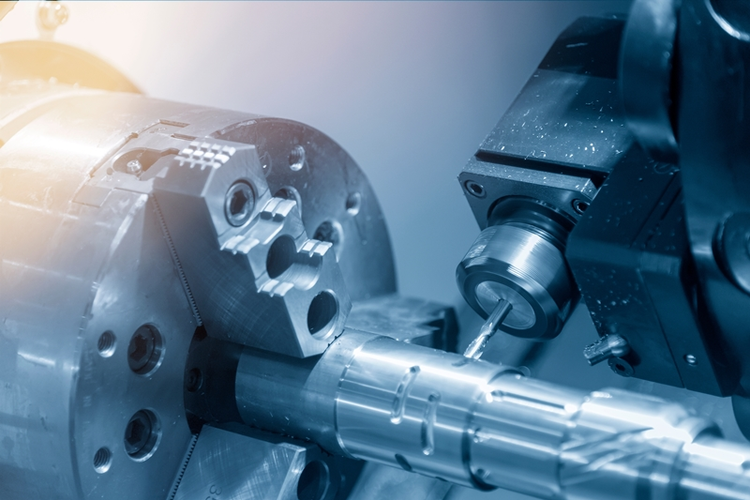The image depicts a close-up view of a CNC machine, likely used in a metalworking or fabricating shop. The machine is actively perforating and detailing a piece of metal, which could either be for shaping a tool or decorating a metal bar. On the right side of the machine, a drill bit is visible, performing the molding and punching tasks. The left side features a cylindrical component with teeth gripping the metal rod, ensuring it is securely held in place during processing. The machine is rendered in a palette of blue, black, and white, with the entire scene suffused with a blue tint and a noticeable yellow glow in the upper left corner of the image.